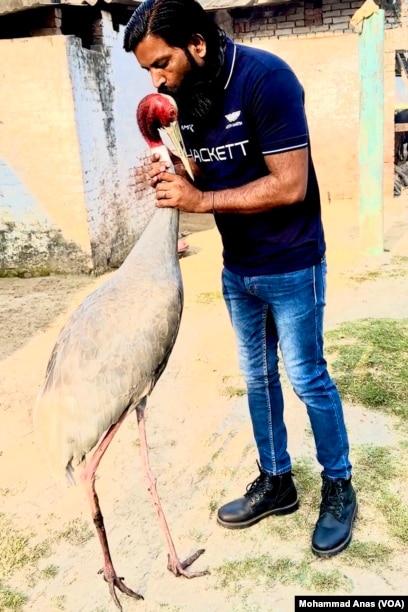In this photograph, an adult male is affectionately kissing the head of a bird. The man, who has dark black skin and a black beard, is dressed in blue denim jeans and a dark blue t-shirt with the caption "HACKETT" partially visible in white. He wears black boots with steel toes. The ground around them is mostly dry, earthy dirt with sparse patches of grass. 

The bird, standing nearly as tall as the man's chin, has a yellow long extended beak and a mostly pink head with slight beige tones on the front. Its body is covered in white feathers with some gray or tan shading, possibly indicating a flamingo or a similar bird. The bird's legs are long and stocky with a mix of pink and brownish-orange hues, turning more brown towards the lower parts.

In the background, there is an old, weathered stone building with some bricks exposed and signs of aging, featuring a mix of white, beige, and brown colors, and some green at the base. The setting appears to be midday, and the atmosphere suggests a serene moment between the man and the bird. In the bottom right-hand corner of the image, there is a black rectangle with the white text "Muhammad and us (V-O-A)". The man seems content and the bird appears to be peacefully enjoying his company.